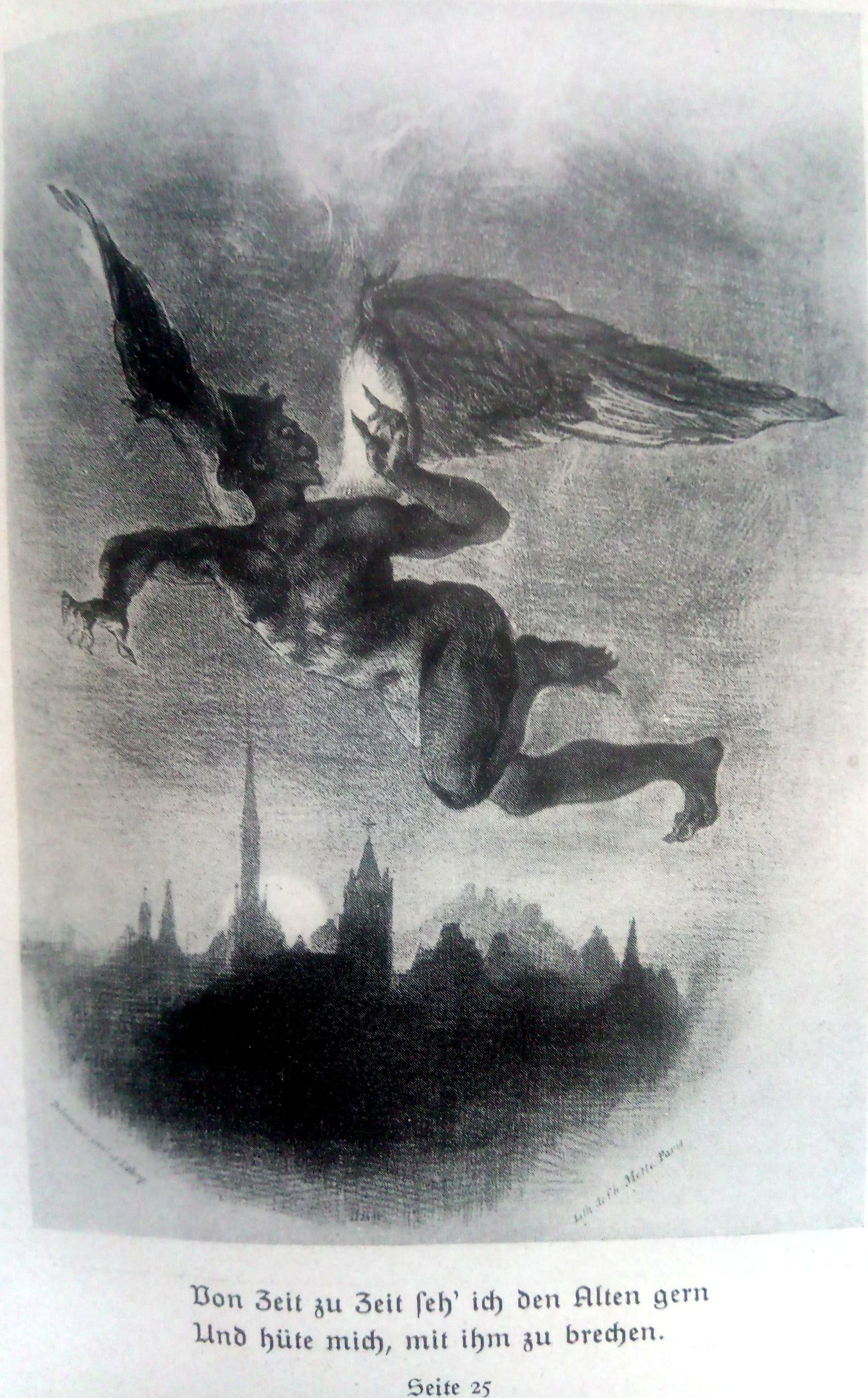The monochrome drawing, evoking a print-like style, portrays a menacing, winged devil occupying the night sky. This muscular, naked figure, characterized by a grotesque, angular face and tentacle-like hands, dominates most of the image. Below, a stark cityscape with spires—likely churches or cathedrals—rises against a mountain backdrop. The scene is rendered in shades of gray and black, with a lighter sky near the horizon. Gothic German lettering beneath the image vaguely reads something akin to "Bonzel Taubeltf Eid. Den Alten Gern Und Hut Emit Ihm Miti Ihm Zu Bredzens Eitie 25," hinting at cryptic or potentially religious messaging. The illustration's setting and composition suggest its origin as a page from a book, possibly containing verse or narrative elements.